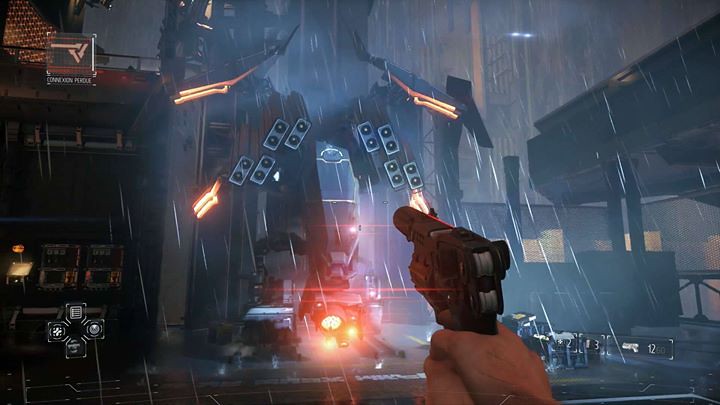A blurred, rain-soaked screen depicts an intense first-person shooter (FPS) video game scene where a colossal mechanical monster devastates a cityscape. Through the lens of the player, clasped hands tightly grip and aim a virtual gun straight at the rampaging giant. This image juxtaposes the chaos wrought by the monster with the player's role, raising provocative questions about the relationship between video game violence and reality. Is the act of aiming a gun merely a harmless in-game action, or does it reflect deeper layers of irony and societal concerns about the impact of video game violence?